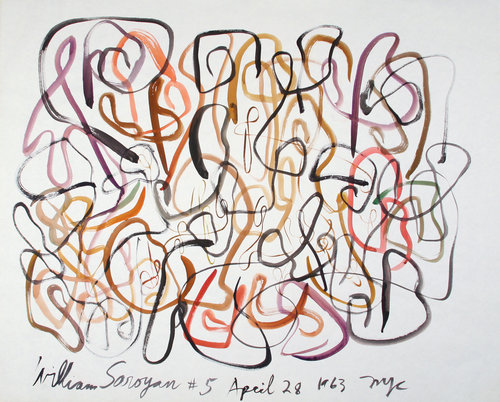The painting features a light gray background covered in an intricate, abstract array of multicolored squiggly lines. The swirling, interconnecting designs are composed of various colors including purple, pink, red, brown, yellow, and black. Some of these lines loosely resemble letters such as B, P, and G, and possibly numbers like 89 and 6, though it's unclear if these shapes are intentional. The overall effect is a vibrant, chaotic mix of patterns that almost seem coded. At the bottom of the canvas, the piece is signed by William Soroyan, dated April 28, 1963, and marked as number 5, with an additional notation that may read "NYC," potentially indicating it was created in New York City. The signature is somewhat difficult to decipher completely.